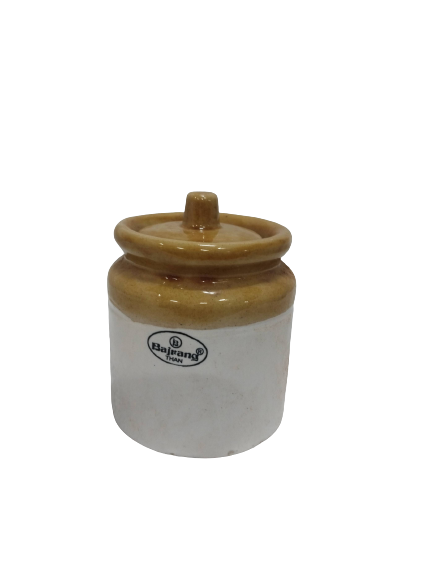This image displays an old-fashioned, ceramic pot placed against a stark white background. The pot, resembling a crock pot or an antique milk jug, features a prominent lid with a round handle at its center, designed for easy lifting. Predominantly gray, the ceramic pot occupies roughly the lower three-quarters of the structure. Midway up this gray section, a black-printed, oval label prominently features the brand name "Bajrang," although the text is slightly obscured. Above the gray ceramic, a glossy light brown accent encircles the upper portion of the pot, seamlessly transitioning into the entirely brown ceramic lid. The entire pot is angled slightly, causing the text and features to be viewed somewhat obliquely, adding a dynamic element to the composition.